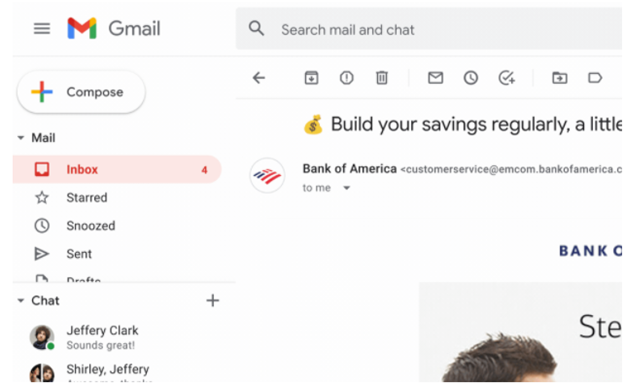The image depicts a user interface, likely from a Gmail application, with various elements organized in a specific layout. 

In the top left corner, a hamburger menu icon is visible, followed by icons and labels in descending order: Gmail, a magnifying glass (representing search), Mail, and Chat. Below these, there are additional icons colored red, yellow, blue, and green, with the label "Compose." 

On the left side, further down the interface, there are icons representing different actions: a trash can, a letter, and a clock. 

In the top left section, "Mail" is prominently displayed. Below this in red text are options such as Inbox, Starred, Snoozed, Sent, and Chat. 

In the messages section, the names "Jeffrey Clark" and "Shirley" are listed. Under Jeffrey Clark's name, the subject "Sounds great" is visible. 

At the top of the interface, there is a highlighted message with a yellow background from Bank of America. The subject reads, "Bill your savings regularly." The message is addressed to the user and mentions "customer service," with the email domain "mcom.com" indicating it’s from Bank of America's customer service.

Also in the interface, there is an image of a person with thick black hair, suggesting a contact or email from a person included in the Gmail previews.